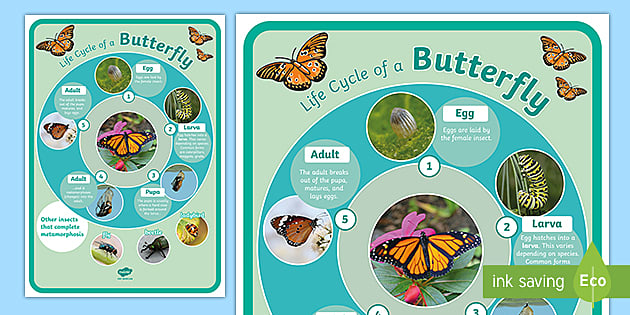The image is an educational poster depicting the life cycle of a butterfly, set against a light blue background. On the left side, the full poster is shown, featuring a prominent title at the top that reads "Life Cycle of a Butterfly" in curved, blue text. Surrounding the title are illustrations of butterflies, specifically two in the upper right corner and one in the upper left, each characterized by their orangish-red wings with black spots and antennae.

The main focal point is a dark blue circle in the middle of the poster, which encircles five numbered stages of the butterfly's life cycle arranged clockwise. Starting from the top, stage 1 showcases the egg, followed by the larva at stage 2, the pupa at stage 3, the adult butterfly at stage 4, and repeated again at stage 5. Each stage is accompanied by a corresponding image to visually depict the transformation process.

On the right side of the image, there is a close-up view of the top portion of the poster. This enlargement highlights the adult butterfly in stage 5, as well as stages 1 (egg) and 2 (larva), providing a clearer look at these sections. Additionally, in the bottom right corner of the entire image, there is a small label in white text with a green border that reads "Ink Saving Eco," with "Eco" encased in a green teardrop shape.